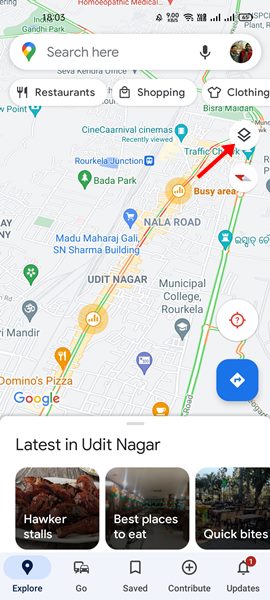The image is a screenshot of a smartphone displaying the Maps application. At the top of the screen is a search bar containing the placeholder text "Search here" in gray, accompanied by a gray microphone icon for voice input. Adjacent to the search bar is a multicolored location dot.

Below the search bar are three interactive ovals. The first oval, labeled "Restaurants," is black and features an icon of a knife and fork. The second oval, labeled "Shopping," displays an icon of a shopping bag. The third oval, labeled "Clothing," contains an icon of a shirt.

The map itself displays various roads, which are color-coded in green and red to possibly indicate traffic conditions. Different location markers are scattered across the map, including a green dot labeled "Bada Park," which has a white tree icon.

At the bottom of the screenshot, there are three descriptive tiles under the heading "Latest in Udit Nagar" written in black text. The left tile reads "Hawker Stalls," the middle tile says "Best Places to Eat," and the right tile is labeled "Quick Bites."

Beneath these tiles are additional icons. The first icon represents a location dot with the label "Explore" underneath it. The second icon is of a car, labeled "Go."